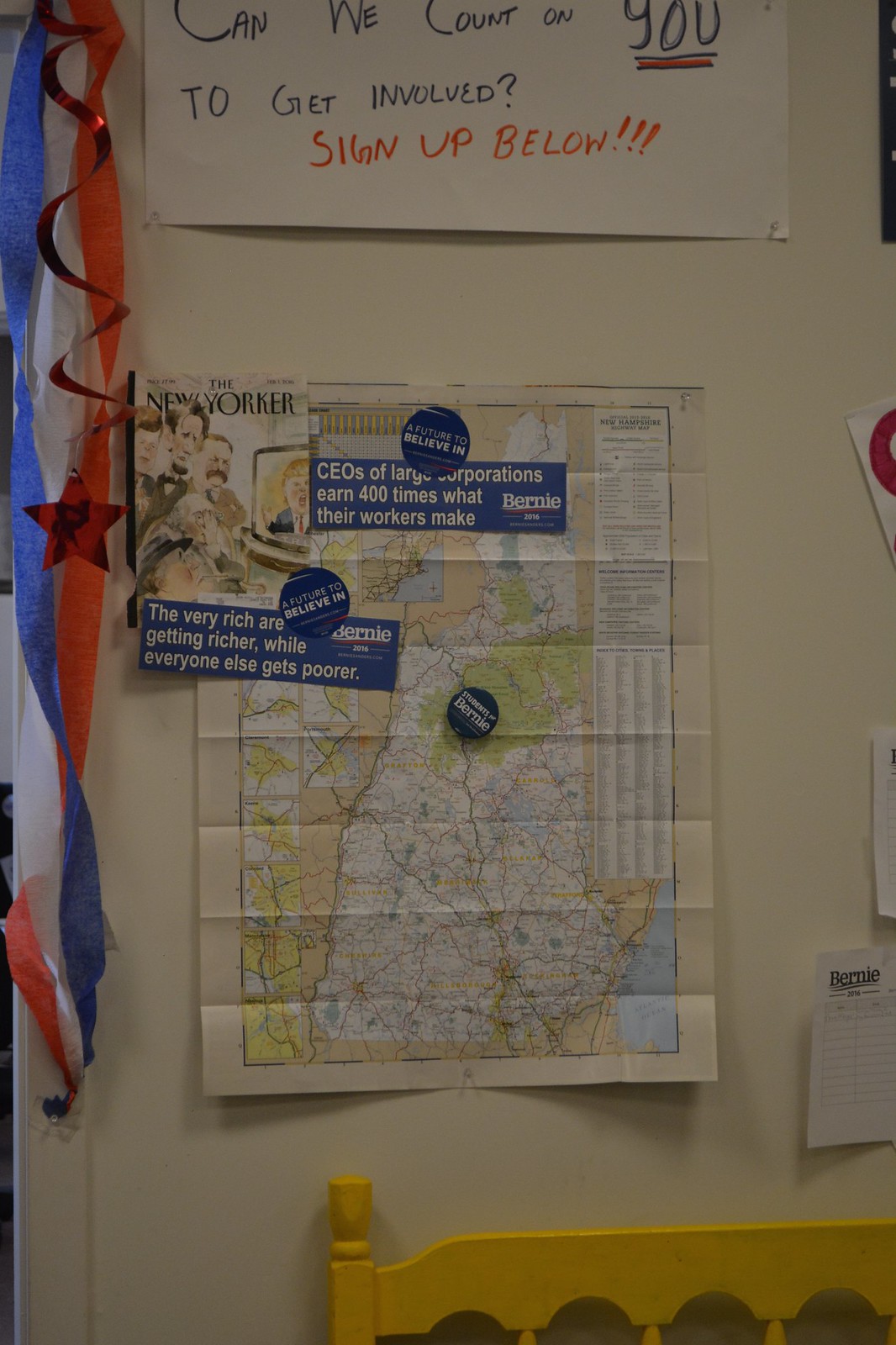The image showcases an indoor setting, possibly a political office or a bedroom based on the tan colored or white wall in the background. Central to the image is a large, unfolded map with various items arranged around it. Above the map is a prominent sign that reads, "Can we count on you to get involved? Sign up below," although there is no sign-up sheet visible beneath it. The map itself features a picture from The New Yorker with the text, “CEOs of large corporations earn 400 times what their workers make. The very rich are getting richer while everyone else gets poorer.” Surrounding the map are several political stickers and pins endorsing Bernie Sanders, including phrases like “A future to believe in” and “Bernie." On the left side of the image, near the top, are red, white, and blue streamers along with a metallic red curl ending in a star. At the bottom of the image, the top of a yellow chair or possibly a headboard is visible. The overall color palette includes shades of red, white, blue, black, gray, yellow, green, and tan.